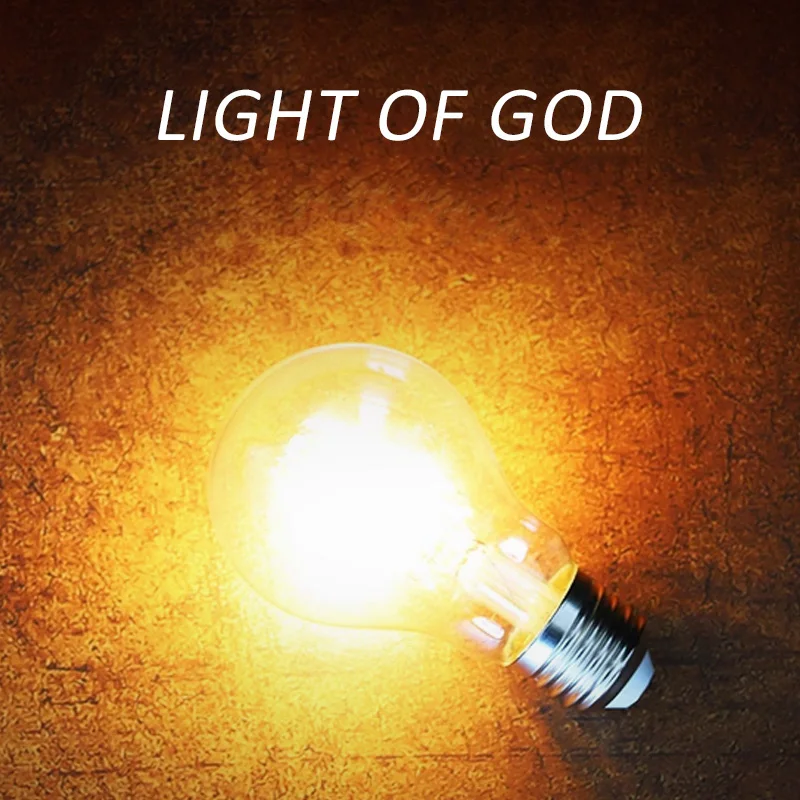This is a square-format color photograph featuring a glowing light bulb at its center. The bulb, with a silver screw base and white tip, emits a bright yellow light from its clear center filament. This illumination creates a radiant glow on the gold mottled background, casting increasingly orange and brown bands as it spreads outward. The lightbulb appears to hover on the surface, without attachment to any socket, suggesting a supernatural element. At the top of the image, the phrase "Light of God" is inscribed in lightweight italic white text. The photograph blends representational realism with text, creating an inspirational visual effect.